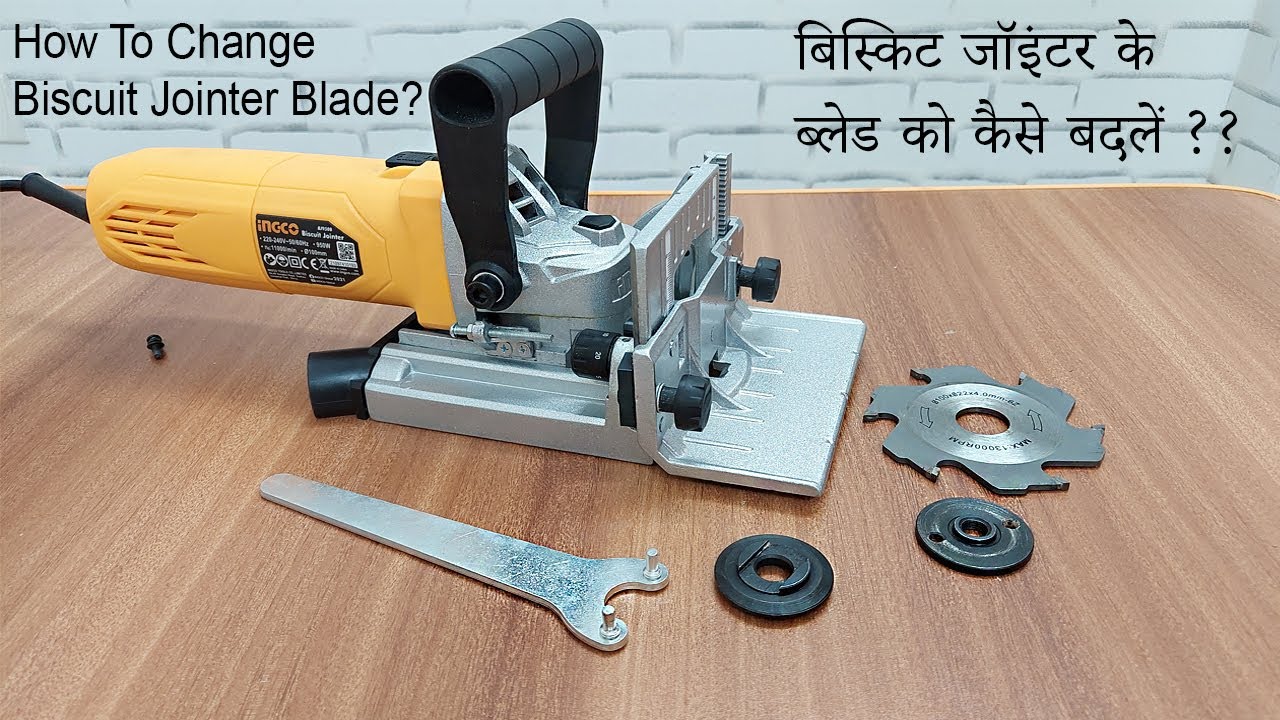The image depicts a large machine prominently featuring a yellow body with a black handle and silver accents, resting on a brown wooden table with a white brick wall in the background. The top left corner includes text that reads, "How to change biscuit jointer blade," although no specific instructions are given. Surrounding the main machine, there are various tools and parts, including a circular silver blade with six points, likely meant for the biscuit jointer, two black circular pieces that seem to secure the blade, and an additional smaller tool, possibly for unscrewing or replacing the blade. The scene also includes a black nail in the background, contributing to the overall assembly of parts related to the jointer. The dominant colors in the image are yellow, black, silver, brown, and white.